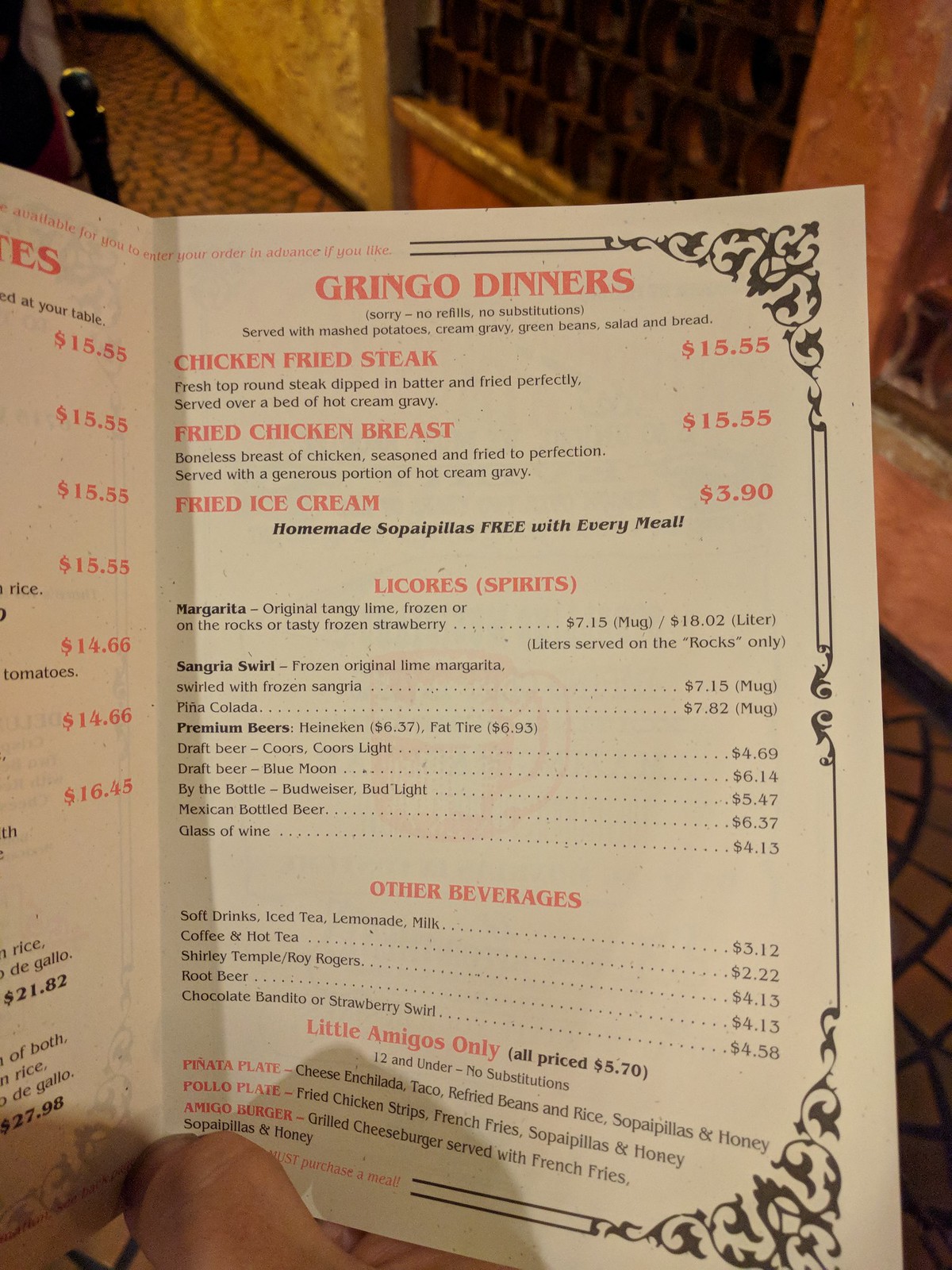Inside a cozy restaurant adorned with white and orange walls and a tiled floor, a patron holds a detailed menu titled "Gringo Dinners." The menu lists a variety of enticing options: Chicken Fried Steak and Fried Chicken Breast both priced at $15.55, and Fried Ice Cream for $3.90. For beverages, it features Liqueur and Spirits including Sangria at $7.15 per mug and Pina Colada at $7.62 per mug. Premium Beers are available at $4.69, with Draft Beer priced at $6.14 and Draft Beer Blue Moon at $5.47. Bottled beer is $5.37, while a glass is $4.15. Soft Drinks are listed at $3.12, Coffee or Tea at $2.22, and specialty drinks like Shirley Temple and Root Beer at $4.15 each. For a sweeter option, there's Chocolate Blendito or Strawberry Swirl at $4.58. The menu also includes a "Little Amiga" section with children's plates.